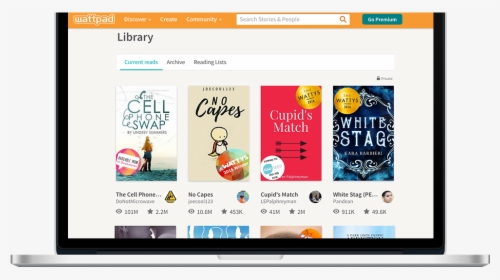In this image, the background is a very light purple, with black framing the sides and bottom edges. An orange banner spans the top of the image. Within this banner, there is a white pad featuring three different toppings, alongside a search bar and a blue "Go" button. Below the banner, the text "Library" is shown underlined, followed by "Custom." Beneath this, there are several books displayed, including titles such as "Sales Swap," "No Capes," "Cupids Match," and "White Stag." Each book listing has a rating indicated by stars and a corresponding prize. The lower portion of the image reveals parts of four more book titles, partially obscured by a wide purple line that stretches across the bottom.